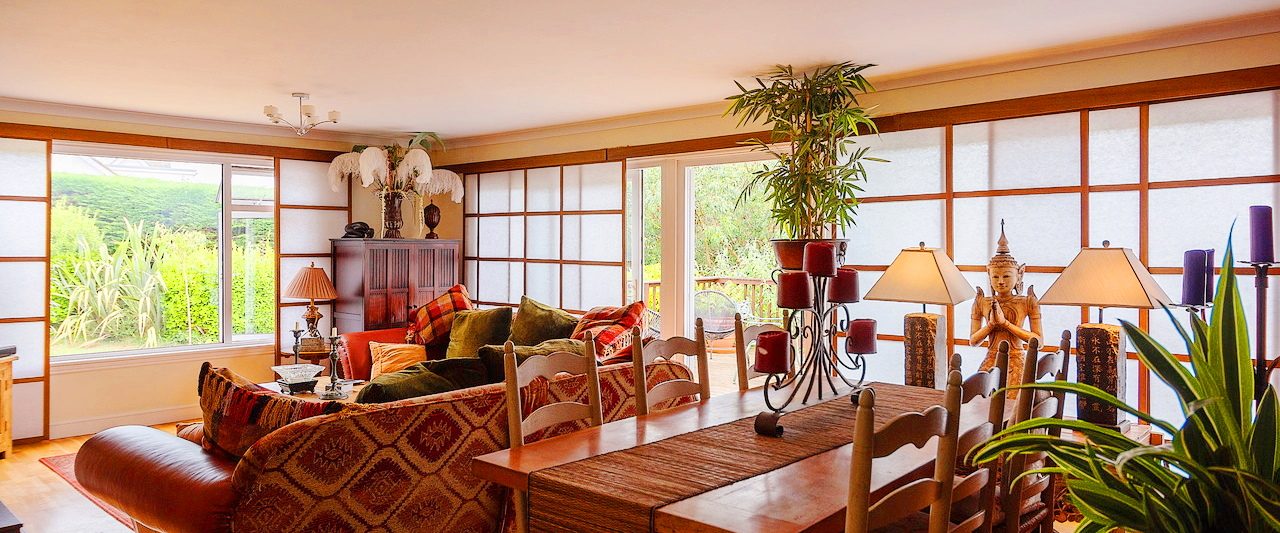This vibrant photograph captures a beautifully decorated living and dining area characterized by warm earthy tones and tropical elements. A warm brown, reddish couch, adorned with red and green pillows and a crocheted blanket, faces away from the viewer towards expansive sliding windows. Outside the windows, lush greenery and a range of mountain vistas hint at a tropical location. Behind the couch, a long dining table with six chairs is set, featuring an elegant candelabrum centerpiece on a table runner. Adjacent to the table stands a serene Buddha statue in a prayer position, flanked by two lamps, adding a touch of spirituality to the room. The foreground is further enriched by plants close to the door and another plant and candles behind the statue, creating an inviting and harmonious atmosphere. In the far corner, a cabinet showcases a vase with plants and feathers along with other sculptural objects, complementing the room's warm and earthy aesthetic.